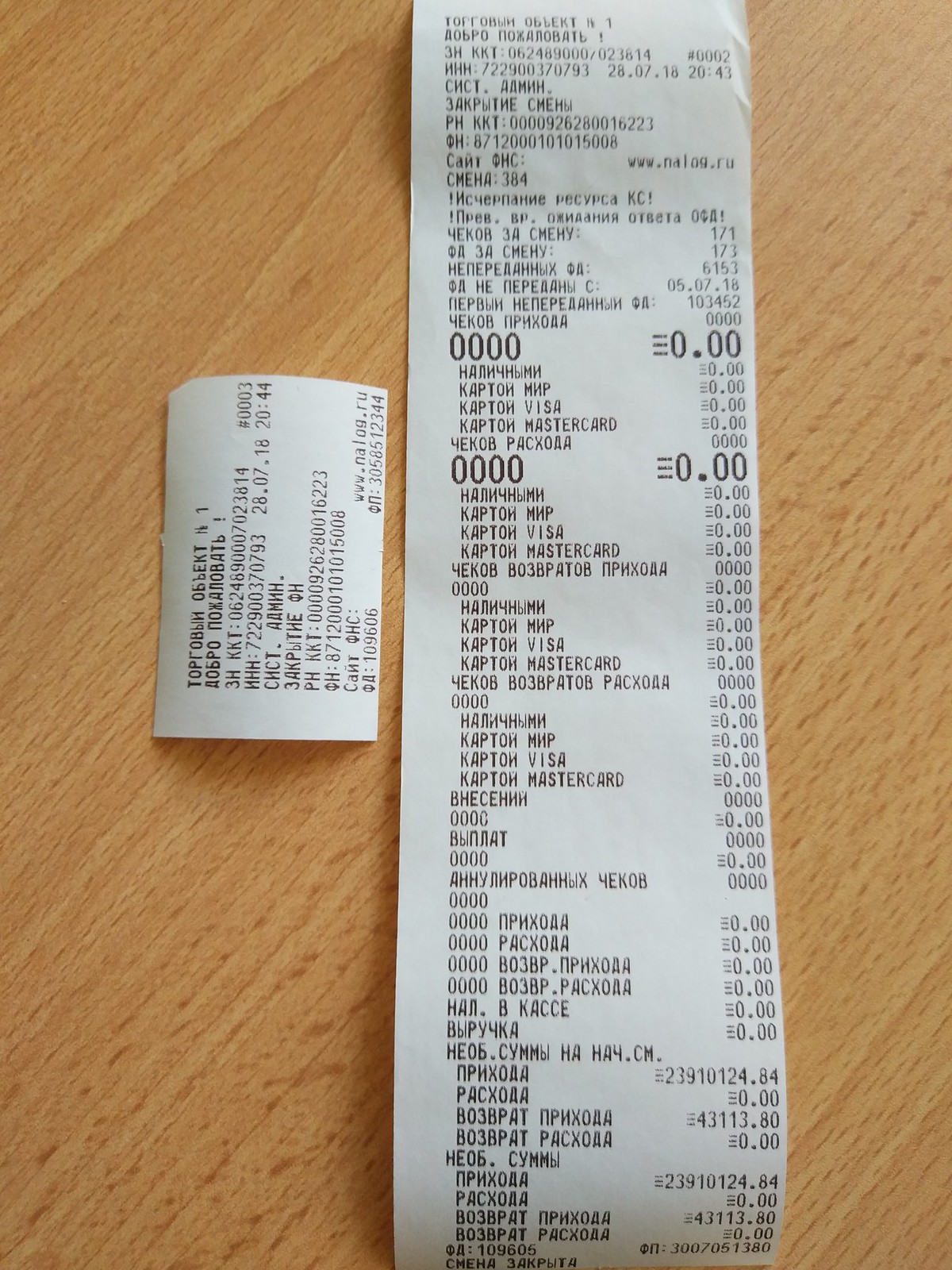This image features two receipts laid out vertically on a light wooden table. On the left side of the photograph, a small receipt is turned sideways, with black text printed on white paper. To its right, centered and occupying most of the image, is a very long receipt with numerous items listed, written in what appears to be Russian. The small receipt is concise, while the large one showcases a sequence of prices, most of which are 0.0000. However, towards the bottom of the larger receipt, there are significant figures listed, including 23910124.84 and 43113.80, repeated multiple times, culminating in an amount of 3007051380 at the very end.